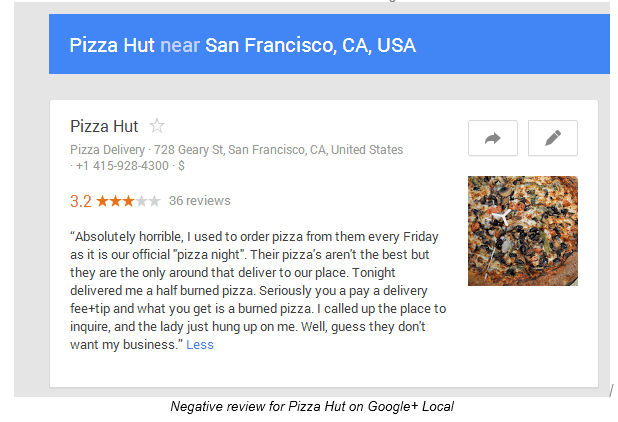The webpage displays information about a Pizza Hut located near San Francisco, California, USA. At the top, a blue bar with white text states, "Pizza Hut near San Francisco, California, USA." Below, on a white background, the text reads "Pizza Hut" alongside an empty white star. The listing includes details such as "Pizza Delivery," the address "728 Gary Street, San Francisco, California, United States," and the phone number "+1 415-928-4300." A gray dollar sign indicates the price range.

The review section features a rating of 3.2 stars, illustrated by three yellow stars and two gray stars, based on 36 reviews. One review criticizes the service: "Absolutely horrible. I used to order pizza from them every Friday night as it is our official pizza night. Their pizzas aren't the best but they are the only around that deliver to our place. Tonight delivered me a half-burned pizza. Seriously, you pay a delivery fee plus tip and what you get is a burned pizza. I called up the place to inquire and the lady just hung up on me. Well, guess they don't want my business." The word "less" appears in blue text, and the review is marked as a "negative review for Pizza Hut on Google Plus local."

There is also an image of a pizza with mushroom toppings, which appears to be burnt.